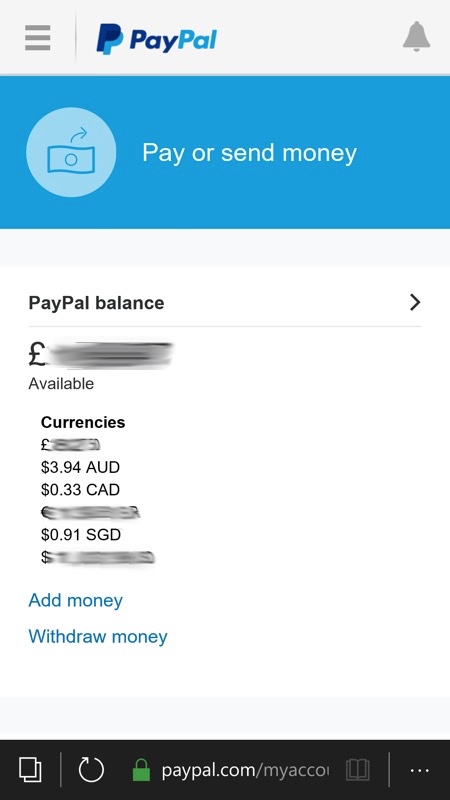The image displays a PayPal webpage. The header of the page is grey, featuring the PayPal logo where "Pay" is in blue and "Pal" is in light blue. The PayPal icon consists of two "P"s, colored blue and light blue, respectively. On the right side of the header, there is a grey bell icon. On the top left, there are three horizontal lines indicating a menu option.

Below the header, there is a blue banner with white text that reads "Pay or send money." Under this banner, the main section shows the PayPal balance. The background of this section is white and the text is black. It displays "PayPal balance," but the actual balance is obscured by a black mosaic for privacy. The section also details "Available currencies," where three currencies are shown, and others are hidden by black mosaic. Specifically, it lists $3.94 AUD (Australian dollars), $0.33 CAD (Canadian dollars), and $0.91 SGD (Singapore dollars).

At the bottom of this section, there are two options in blue text: "Add money" and "Withdraw money." Below this, in the footer of the webpage, there is a tab menu with icons and options labeled as "Reload," "Unlock," and "PayPal.com." The section also includes "My account," written in white.